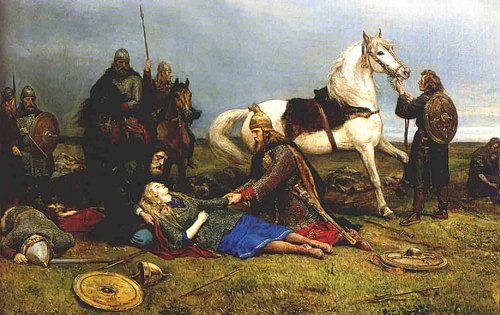The painting depicts a somber scene in the aftermath of a medieval battle. At the center lies a woman, prostrate on the ground, clad in a gray overcoat, a blue skirt, and maroonish boots or stockings. Her head is gently cradled by an elderly man, hinting at her imminent death. A younger man, distinguished by his gold helmet and heavy velvet coat, kneels by her side, holding her hand. His sword is still sheathed at his side, and a helmet is discarded on the ground nearby.

In the background, a white horse with a black saddle is calmed by a man, while other heavily armored warriors, some on horseback and some on foot, loom behind. One such soldier, with a shield on his back, appears to be providing guidance. Off to the side, three men stand apart, seemingly indifferent to the woman's plight. The air is heavy with sorrow, emphasized by the gray, gloomy sky overhead and the battle-worn grass underfoot. Nearby, another warrior lies face down, most certainly dead, with his sword and helmet still intact. The bronze shields present in the scene and the splashes of red on the soldiers' clothing contribute to the grim, melancholic mood of the painting, conveying the dire cost of the conflict.